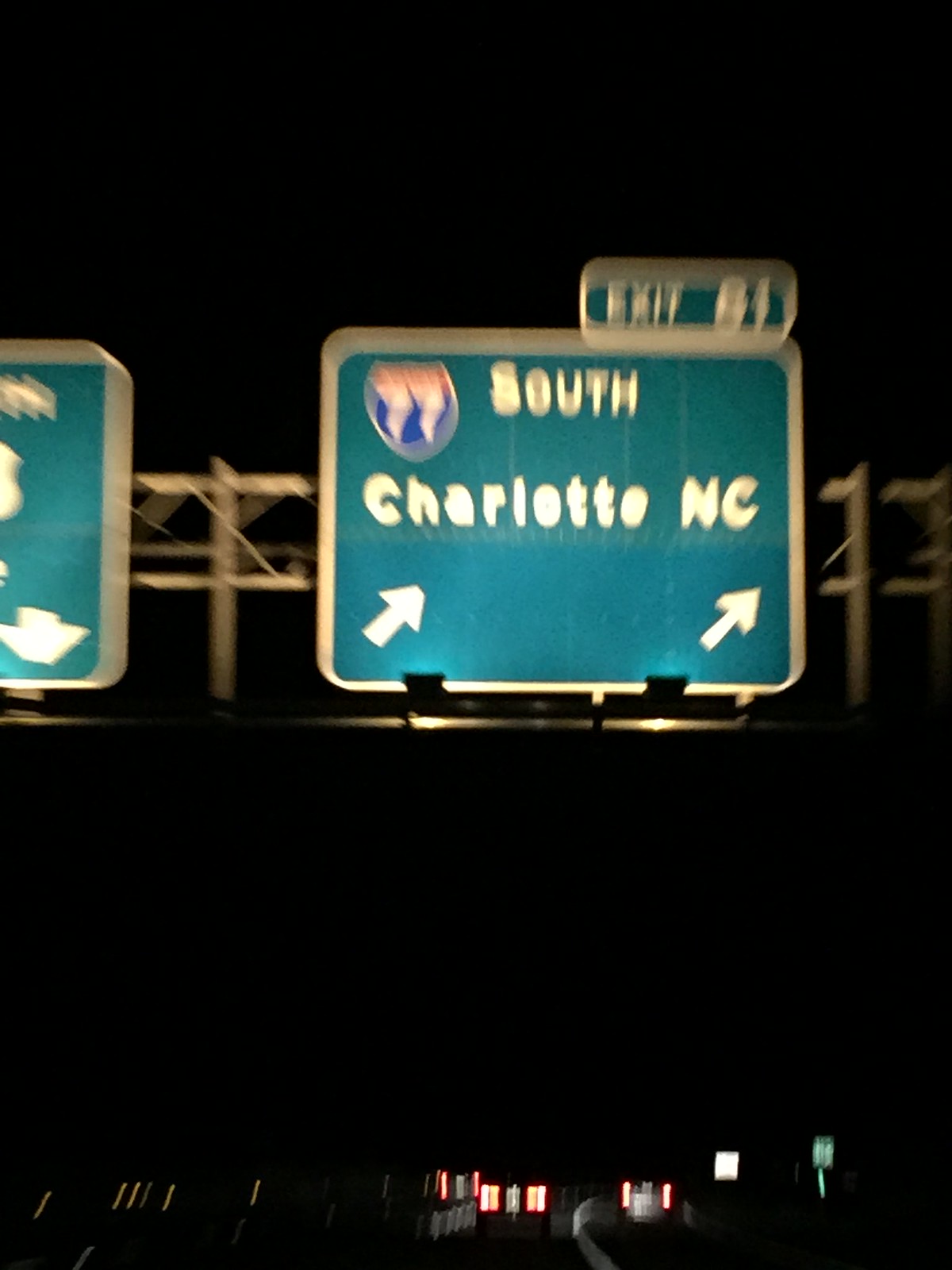This nighttime photograph, likely captured from the front windshield or a dashboard camera of a moving vehicle, shows a scene on a busy expressway. The image, though blurry, depicts several lanes filled with cars traveling in the same direction, their red taillights creating streaks of light in the dim setting. Overhead, multiple directional signs are visible, one prominently indicating "77 South Charlotte North Carolina" with arrows pointing to the right, suggesting an exit to the right. The exit number on the sign is indistinct and appears to be either 61 or 81, adding to the impression of motion and speed captured in this drive-by shot.